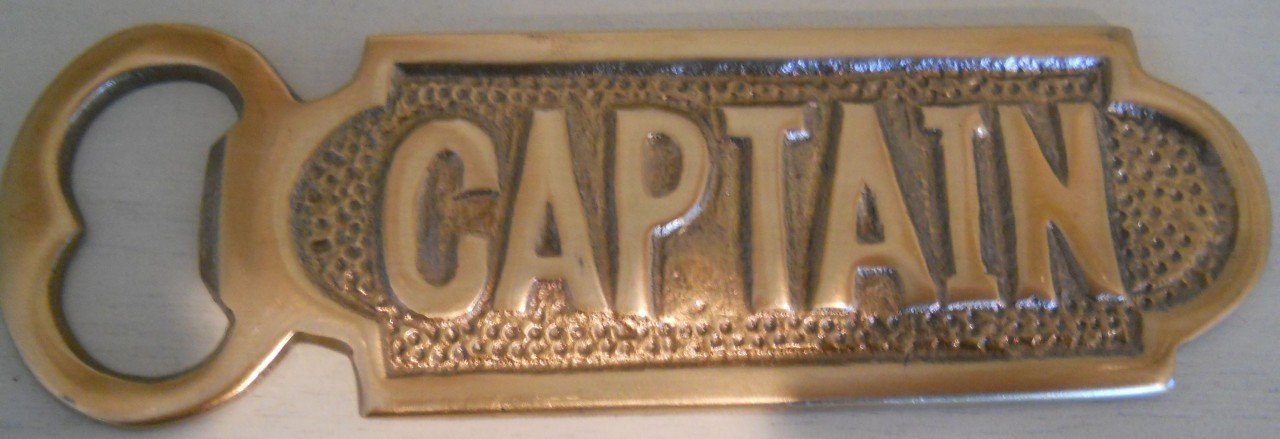The photograph depicts a brass-colored, manual bottle opener with a distinct and intricate design. The opener is placed on a light gray, wood-grained surface. The main body of the opener is rectangular with semi-circular extensions on both the left and right sides. Prominently engraved in raised lettering in the center of the opener is the word "CAPTAIN," surrounded by small indented dots. The rectangular shape is encased within a thin border that traces the perimeter. The left side of the opener features a shiny metal mechanism for removing bottle caps, resembling a pit scoop with a round double circle shape and a small slanted end.